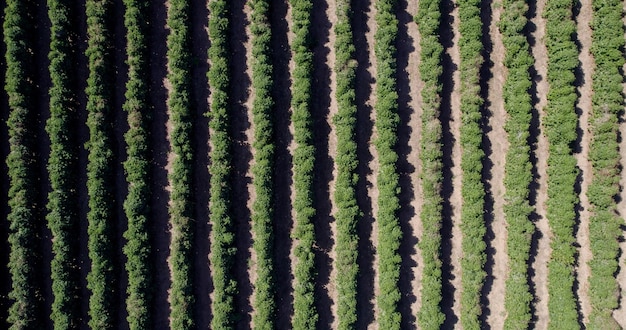This aerial landscape image, likely captured by a drone or helicopter, showcases a farm with meticulously organized rows of dense green vegetation, possibly an orchard. The rows of plants are perfectly parallel, stretching vertically from the top to bottom of the photograph. Between each row, the brown soil is visible, creating clear separations where one could walk. The plants are uniformly arranged, suggesting careful cultivation, but the specific type of plant is not identifiable. Bathed in sunlight, the photograph reveals that the light source is coming from the left, casting pronounced shadows that fade from left to right. As a result, the left side of the image appears darker with less visible soil, while the right side is brighter, allowing a clearer view of the light-brown earth between the rows.